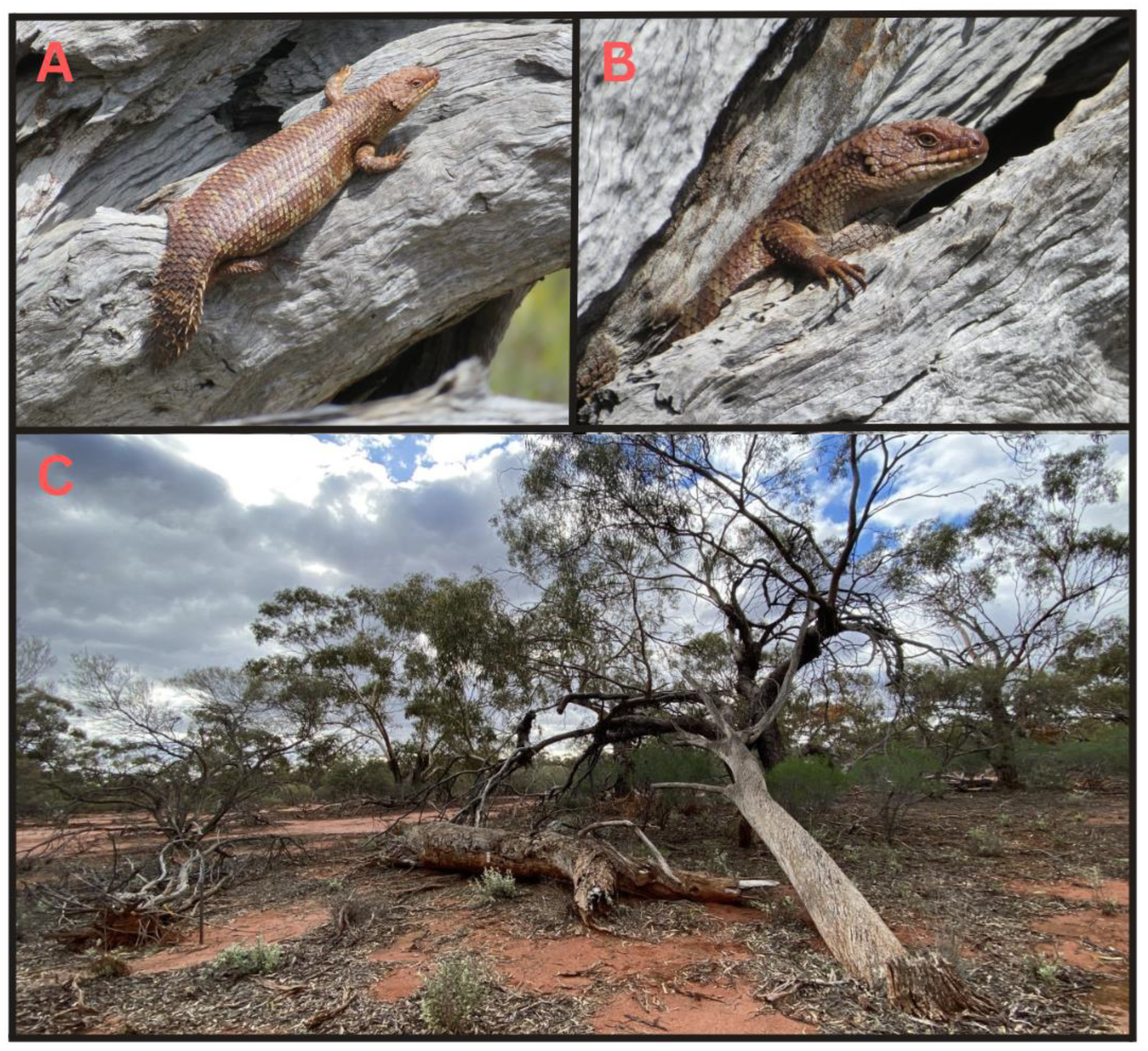This image consists of three color photographs, labeled A, B, and C in red text at the top left corner of each photo. The two upper images (A and B) are side-by-side and of equal size, while the bottom image (C) is larger and spans the same width as the two above. In photograph A, a brown lizard is seen crawling on a gray tree limb, with a rounded belly and short blunt tail, facing the top right. Photograph B offers a close-up profile of the lizard’s face, partially hiding among branches. The bottom photograph (C) presents a wider landscape view, depicting the lizard's sandy, reddish-brown dirt habitat with scattered branches, rubble, and green trees on the horizon. Overall, the images come together to provide a detailed representation of the lizard and its natural environment under a blue sky with some clouds.